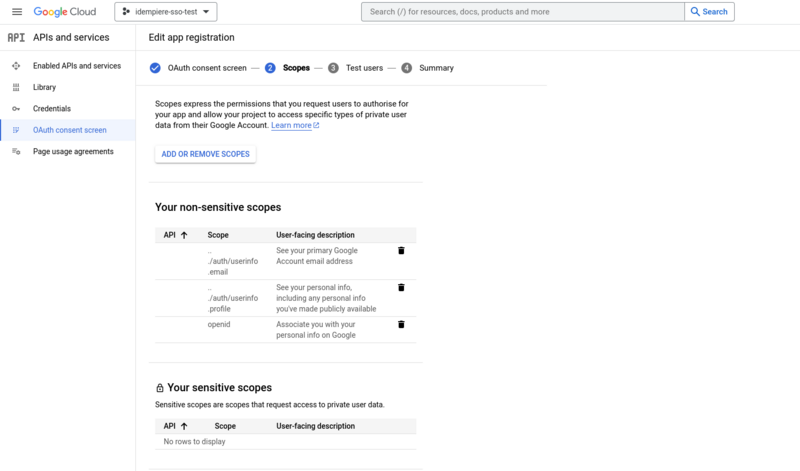This image depicts a screenshot of the Google Cloud interface in landscape orientation, clearly designed for a computer or laptop display and set against a plain white background. At the top of the interface, a black hamburger menu icon is displayed on the far left, followed by the Google logo with the word "Cloud" next to it. Adjacent to this, a drop-down box labeled "ID and peer SSO test" is situated. Moving further right, there is a gray search box with placeholder text in grayish font, and a white box featuring blue text that reads "Search."

Below this top row, on the left-hand side, a column titled "APIs & Services" displays several options: "Enabled APIs & Services," "Library," "Credentials," "OAuth Consent Screen," and "Page Usage Agreements." Dominating the rest of the page is a section with the header "Edit App Registration." This section includes a blue circle with a white check mark indicating the "OAuth Consent Screen," followed by navigation pathways and a white box with a blue font button labeled "Add or Remove Scopes."

Further down, the interface is divided into sections for managing scopes. The "Your Non-Sensitive Scopes" section is marked with a black text header over a white background and features a gray box with black font labeled "API Scope User Facing Description," alongside a white box with miscellaneous icons. Below this, a lock icon denotes the "Your Sensitive Scopes" section, signifying areas requiring additional security or permissions.